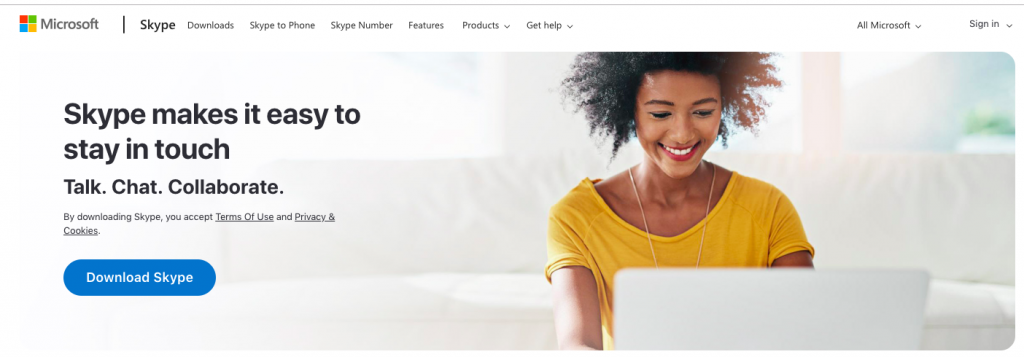This image appears to be a promotional page for Skype on Microsoft's website. Set against a clean white background, the layout features a navigation bar at the top. On the far left of the navigation bar, there is the Microsoft logo—a large square composed of four smaller squares in red, green, blue, and yellow. To the right of the logo, a series of menu options are displayed, reading from left to right: Skype, Downloads, Skype to Phone, Skype Number, Features, Products, Get Help, All Microsoft, and Sign In. The last four menu options include down arrows, indicating dropdown menus for more options.

Below the navigation bar, there is a bold black text slogan: "Skype makes it easy to stay in touch, talk, chat, collaborate." Further down, it mentions that by downloading Skype, users accept the terms of use and privacy and cookies policies, both of which are hyperlinked.

Prominently featured below this text is a blue button with white lettering that says "Download Skype." Adjacent to this button is a captivating image of a Black woman who is smiling down at her laptop. She is adorned with bright red lipstick, an afro hairstyle, and is dressed in a yellow shirt and a gold necklace. She is seated on a white couch, intently engaged with her silver laptop. In the far background, windows provide a glimpse of natural light, and off to the far right, a small green blur suggests the presence of a plant.